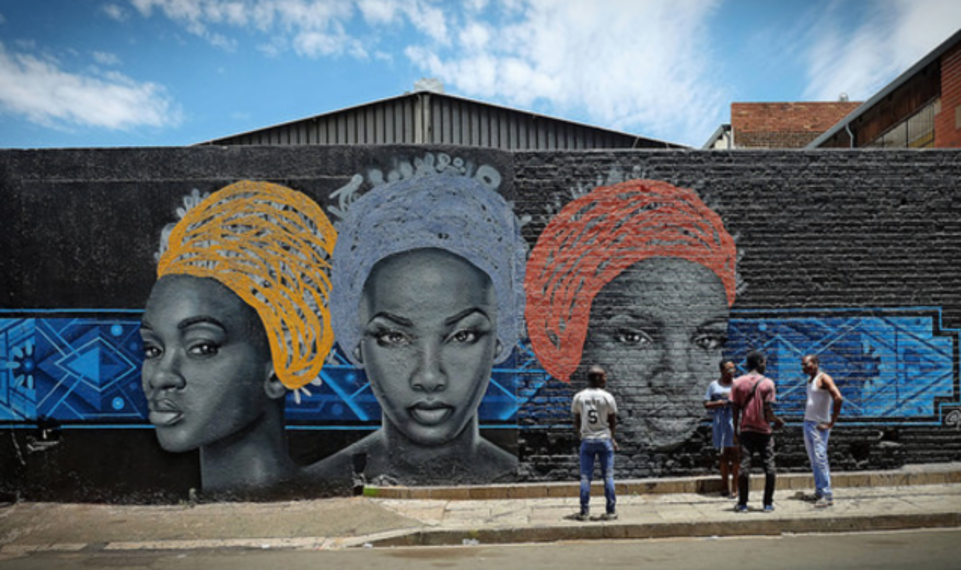The photograph features a striking mural painted on a large, dark black wall, part of a setting that includes a gray sheet metal building in the background and adjacent red and brown brick buildings with clear front windows. The mural itself portrays three African-American women adorned in African-style headdresses— the one on the left wears a yellow headdress, the center woman a cyan headdress, and the woman on the right a red headdress. Each woman gazes thoughtfully: the left one looks to the side, the center one gazes straight ahead, and the right one looks slightly downcast. Behind them is a decorative embordered rectangle filled with a geometric motif comprising various shades of blue diamonds and circles. In front of the mural, four African-American men stand on a beige-colored sidewalk. One man, wearing a white tank top and blue jeans with brown shoes, stands with two others who are dressed in a short-sleeved red T-shirt and dark jeans, and a long-waisted T-shirt with dark shorts. Another man, sporting a white shirt with the number five in black, blue jeans, and white shoes, stands apart from the group, seemingly observing the artwork. The scene is completed with a bright blue sky dotted with soft, white puffy clouds above.